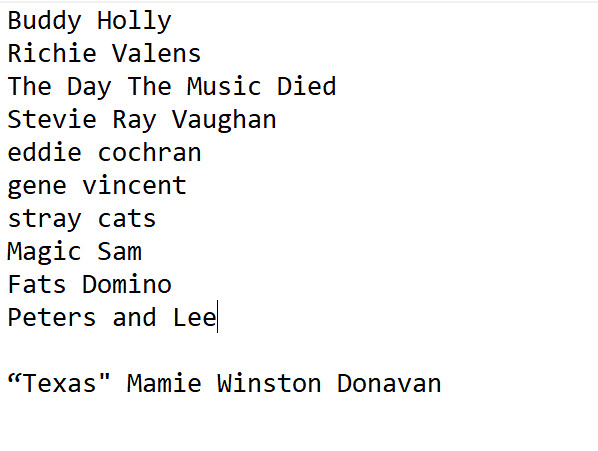The image features a list of musical artists and song names set against a completely white background. The text is black and positioned along the left side of the image, taking up most of the space in a portrait orientation. Each name is presented on a separate line in a typewriter-style font. The list includes the following in order from top to bottom: Buddy Holly, Richie Valens, The Day the Music Died, Stevie Ray Vaughan, Eddie Cochran, Gene Vincent, Stray Cats, Magic Sam, Fats Domino, Peters and Lee, "Texas" Mamie Winston Donovan. The simple and clean design suggests a typographic graphic style, reminiscent of text on a piece of paper or a sticky note, with the sole focus on highlighting the names of these musicians.